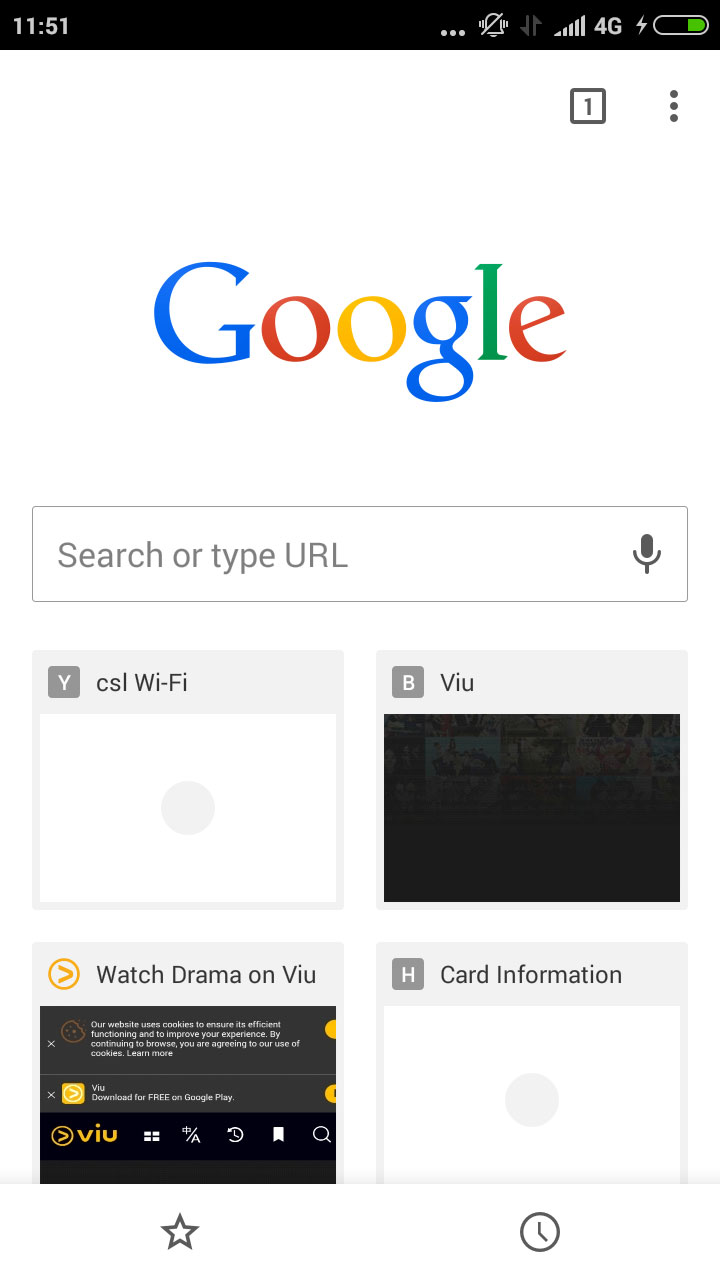The image is a vertical screenshot of a cell phone screen, approximately twice as tall as it is wide. At the very top, a black status bar spans from left to right, displaying the time, 11:51, on the upper left. To the right, various icons indicate signal strength and battery level.

Beneath this bar, there is a browser interface with one open tab, indicated by a small box containing the number 1 and an adjacent three-dot menu icon on the upper right.

The homepage loaded on the screen is Google's, prominently featuring the Google logo in its familiar colors: blue, red, yellow, blue, green, and red letters centered at the top of the view. Midway down the screen, about 40-50% of the way, sits a search bar with the text "search or type URL" displayed in gray, accompanied by a black microphone icon on the right for voice input.

Below the search bar, four suggested websites are listed. The first link is to "CSL Wi-Fi," followed by "VIU" and "Watch Drama on VIU." The final link, titled "card information," is situated towards the lower right of the screen.